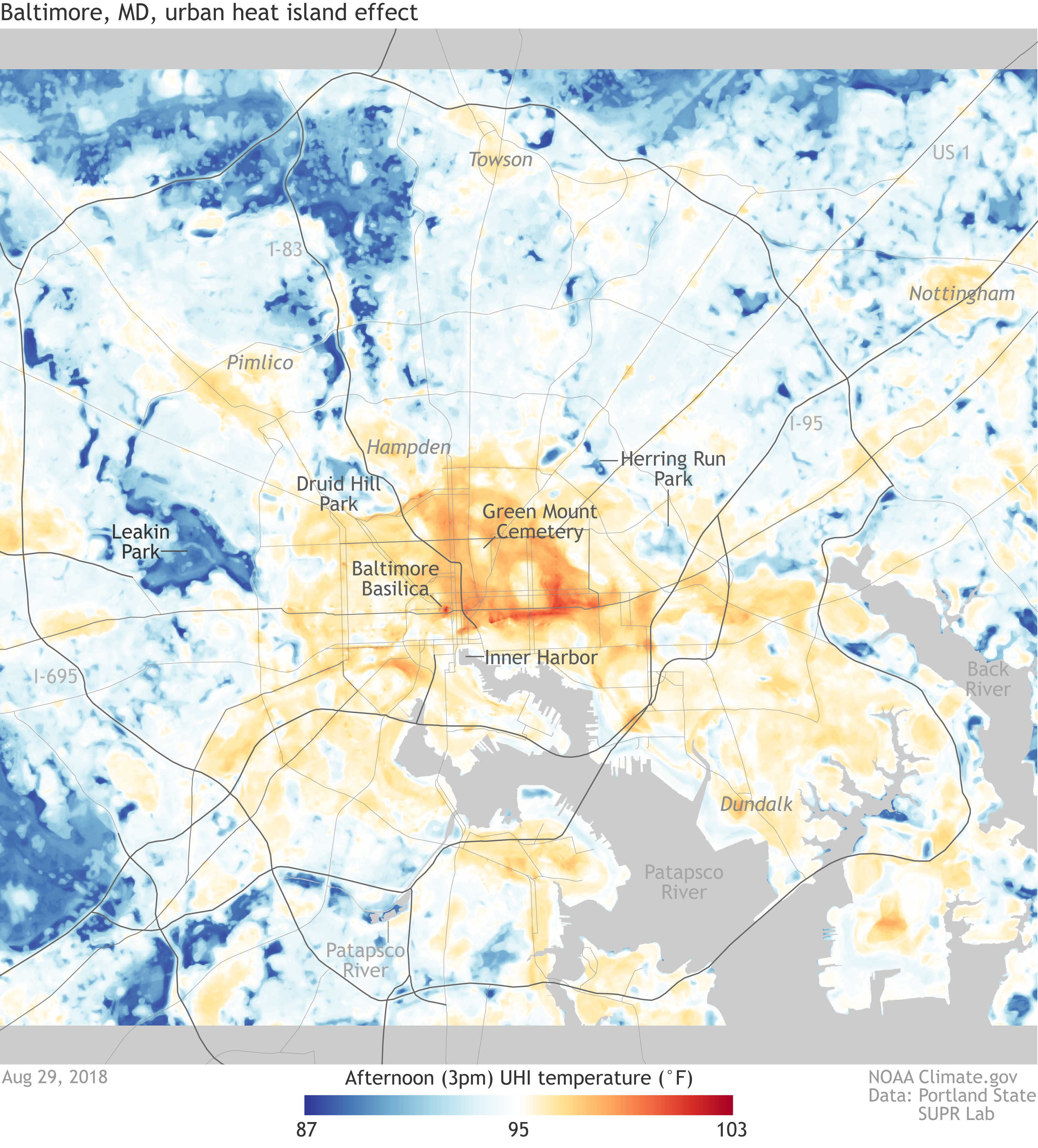The image is a detailed heat map titled "Baltimore, Maryland Urban Heat Island Effect," with data sourced from NOAA climate.gov and Portland State SUPR lab, dated August 29th, 2018. Central to the image is a color-coded graph depicting afternoon temperatures at 3 p.m., ranging from 87°F to 103°F using a gradient from blue to red. The cooler outskirts of Baltimore, like Nottingham and Herring Run Park, show temperatures around 87°F (blue), while central urban areas such as Baltimore Basilica, Green Mount Cemetery, and Inner Harbor exhibit much higher temperatures nearing 100°F (red). Additionally, white spots on the map indicate regions with approximately 95°F, highlighting the significant variations in heat across different areas.